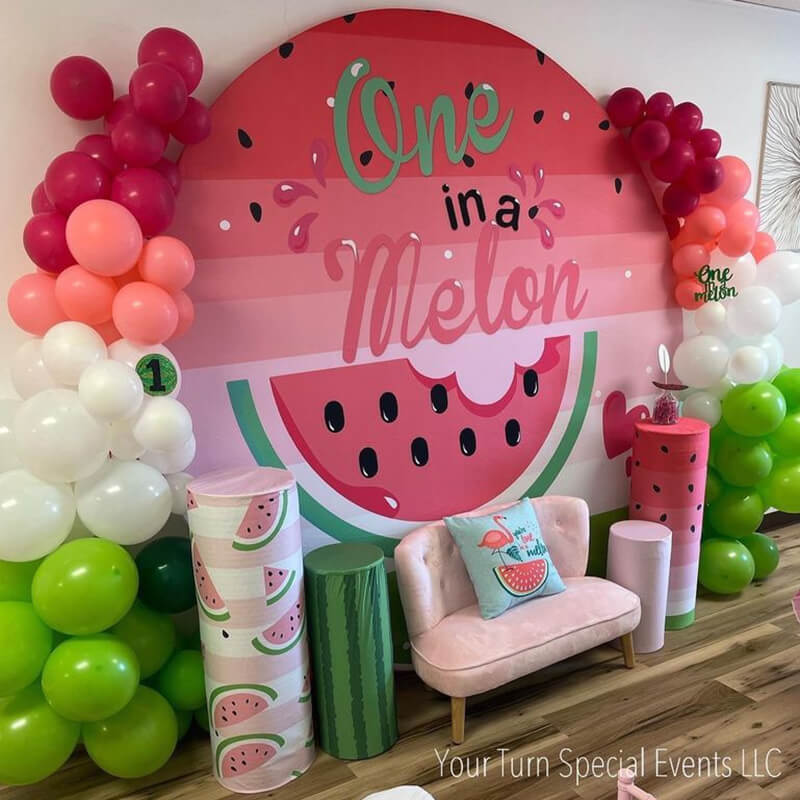The image depicts a vibrant, watermelon-themed birthday party setup. Dominating the scene is a gigantic circular sign with the cursive text "one in a melon," featuring "one" in green and "melon" in pink, complete with a watermelon slice illustration beneath it, complete with black seeds, and green, white, and pink layers. This sign is mounted against a large, white wall and is surrounded by an eye-catching array of balloons in various colors, including green, pink, yellow, and white, reminiscent of a watermelon's hues.

Below the sign is a pink bench adorned with a blue pillow, which is decorated with a flamingo and a watermelon, adding a playful touch. On either side of the bench stand four vertical posts, each with distinct watermelon-themed decorations: one is entirely green, another predominantly pink, and others feature layers mimicking the watermelon pattern. A black number "1" is visible on the left side, placed on one of the white balloons with a green background, indicating the celebration of a first birthday. The flooring beneath the setup is brown vinyl, complementing the vivid decorations and adding warmth to the festive scene.